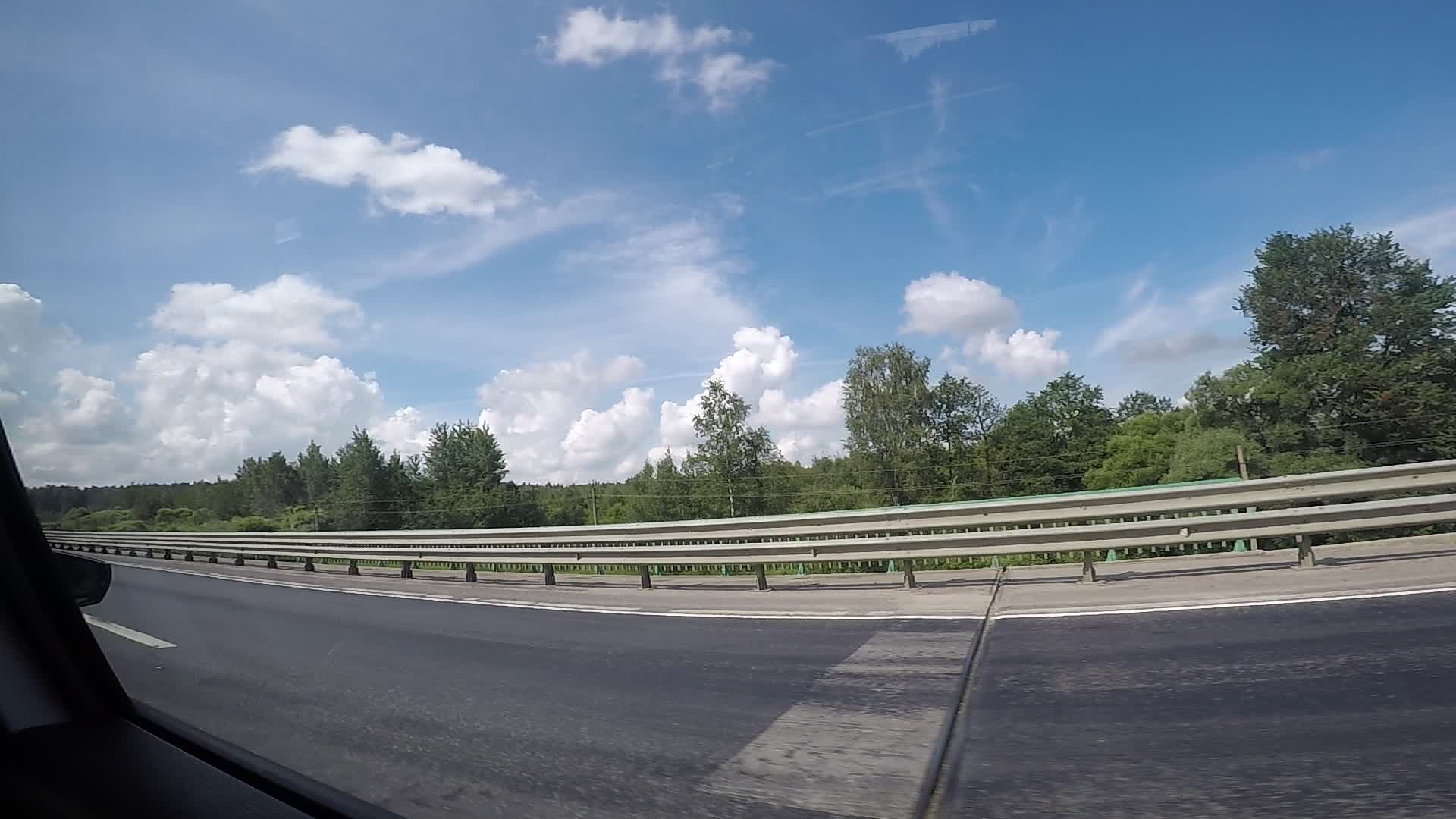A clear blue sky dotted with multiple fluffy white clouds stretches overhead. Below, a row of tall trees stands proudly, their lush green leaves forming a vibrant canopy across the middle of the scene. In the foreground, a sleek railing runs parallel to a black asphalt pathway, which features a prominent white line dividing it down the center. The background fades into a softer gray, providing a subtle contrast to the vivid colors of the foreground elements.